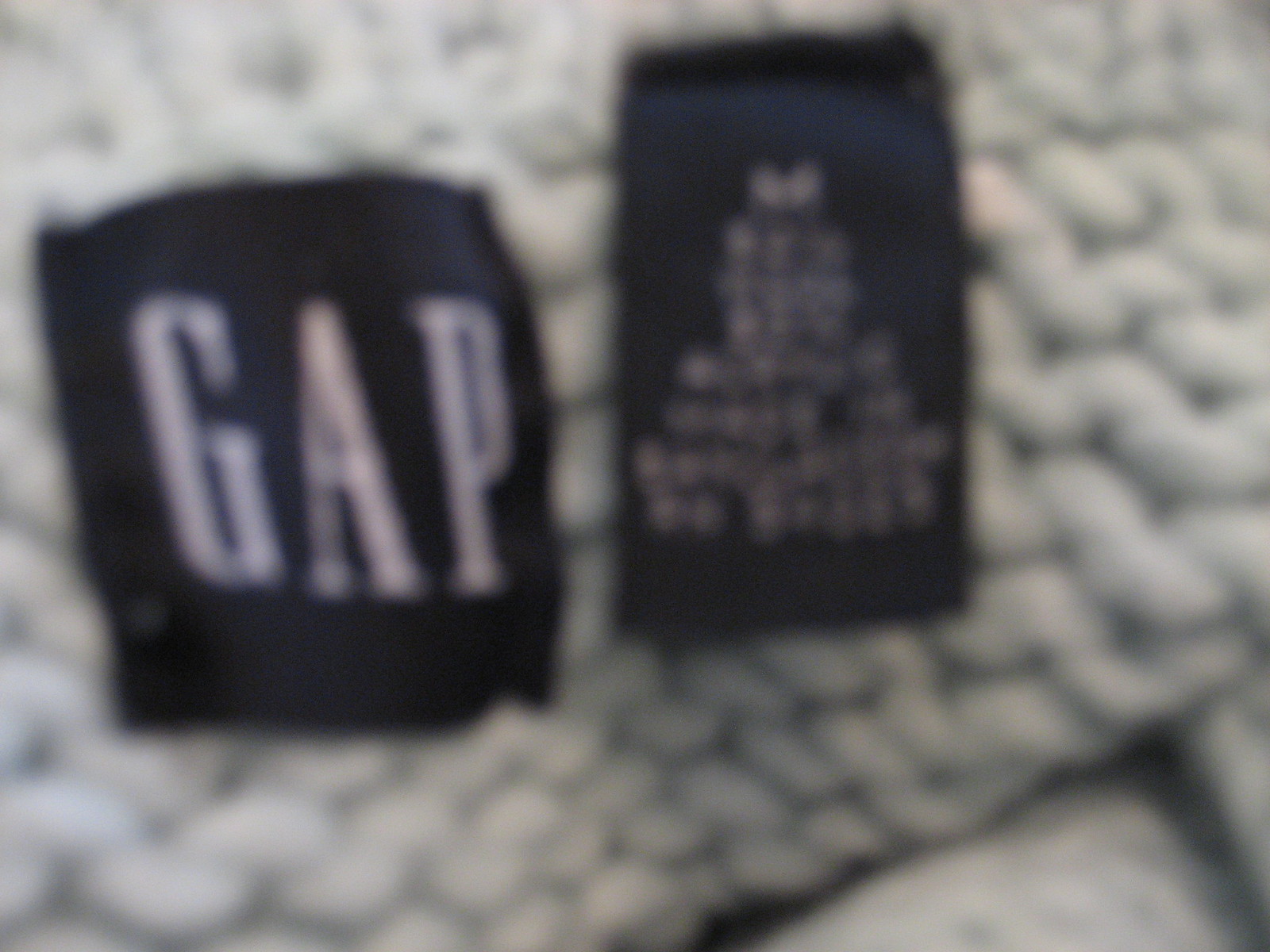A heavily zoomed-in and very blurry image shows two tags attached to a piece of fabric, possibly clothing or a blanket. One tag, a square-shaped black label with bold white "GAP" lettering, is prominently visible. The other, a vertical rectangle tag featuring a lot of small white text, is too blurry to read but hints at providing care instructions and material information. The fabric appears gray and woolen, suggesting it might be the inner lining of a coat, a shirt, or a cardigan. The image is of poor quality and lacks clarity, but it clearly identifies the garment as a GAP product.